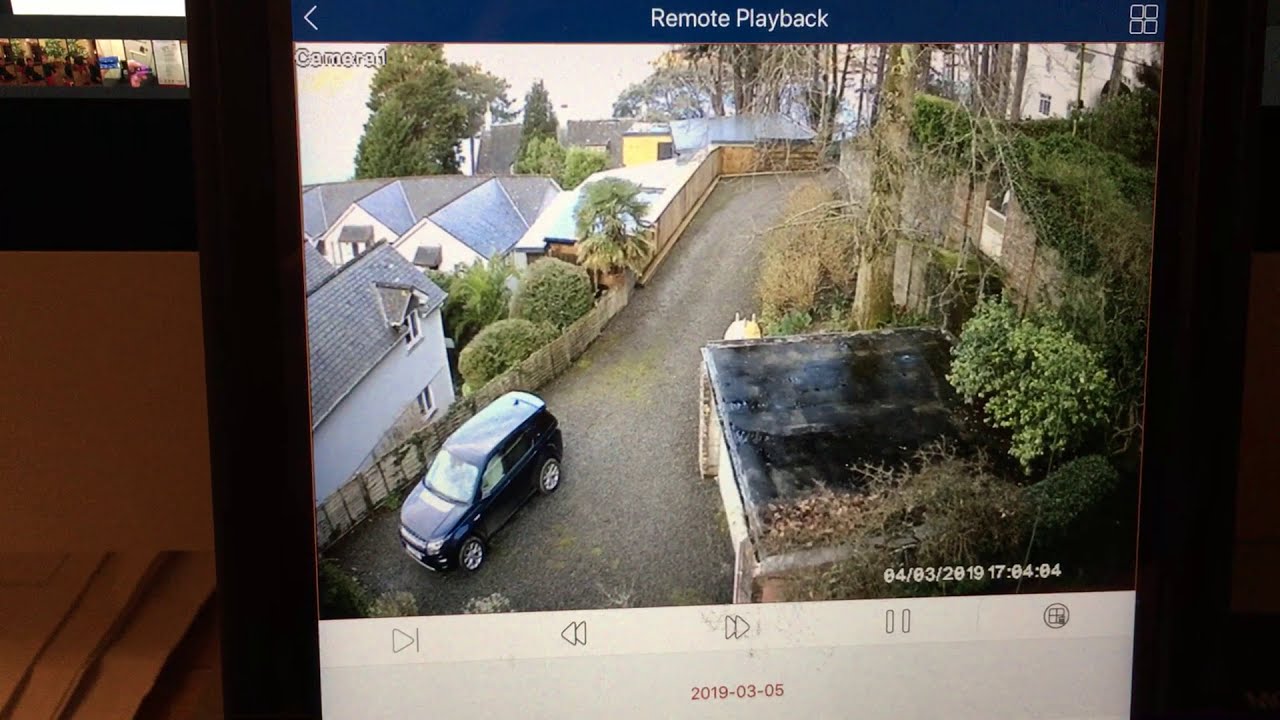The image is a detailed screenshot of security camera footage displayed on a monitor. At the top, a blue horizontal strip with white text reads "Remote Playback." The imagery appears captured from a high-mounted surveillance camera, showing a compact residential area with interconnected white and gray houses, characterized by numerous trees, shrubs, and a narrow asphalt road. A blue SUV is parked nearby, just outside a small garage overgrown with vines and brush. The screen displays familiar playback controls—play, rewind, fast forward, and pause—along with a date, "2019-03-05," in red font. Additionally, there is a "Camera 1" label on the screen's left, and the time "17:04:04" is indicated at the bottom-right corner. The layout suggests the image might be seen on a tablet, capturing a moment from the surveillance footage of this foreign-looking neighborhood.